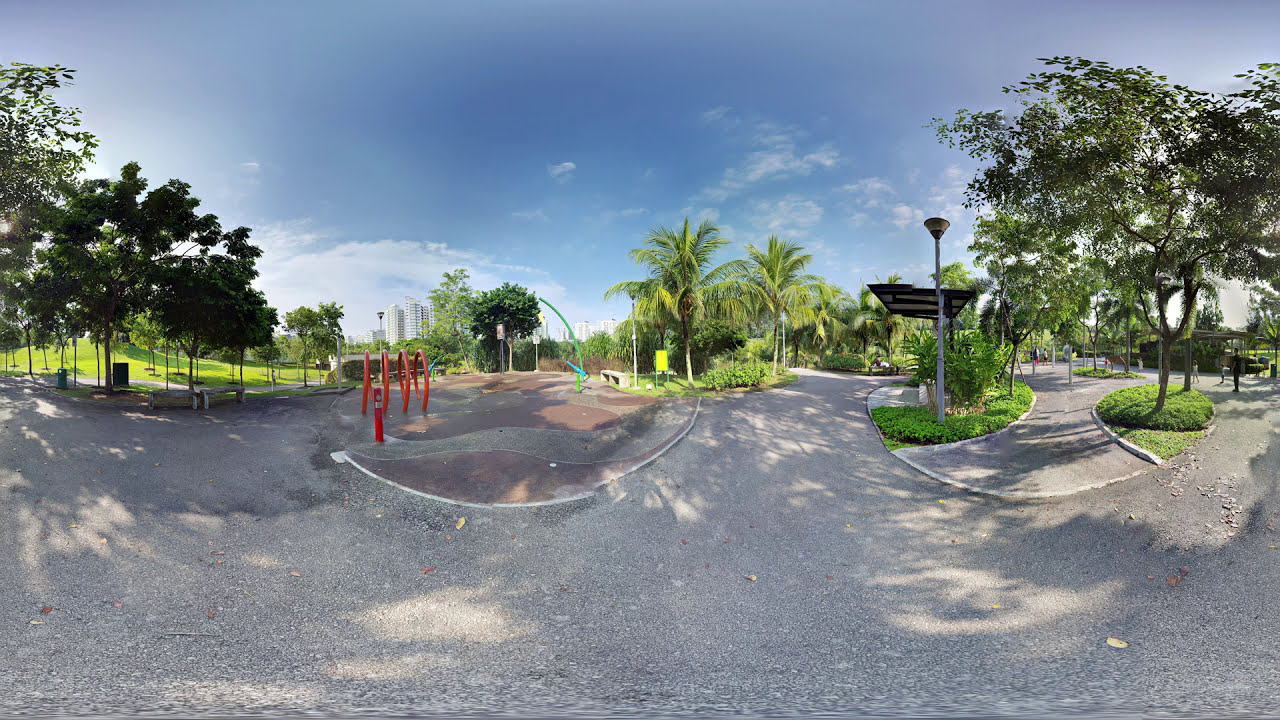This detailed fisheye lens panoramic image showcases an expansive suburban park on a bright and sunny day. In the mid-left of the image, four interconnected orange poles curve to form playful loops, likely crafting a unique playground structure. Adjacent to this, to the right, stands a vibrant green and blue contraption, further hinting at the playful nature of this area. The scene is enriched with palm trees that punctuate the background, suggesting a warm, summery climate. The park’s landscape features a mix of loose rock and slightly paved gravel pathways that branch out in multiple directions, dotted with some dirt, rocks, and scattered leaves. Decorative brown signposts with yellow inscriptions and strategically placed orange cones are also visible along these paths.

The setting is framed by a wide blue sky with a scattering of wispy white clouds. Notably, the park is devoid of people, amplifying its serene ambiance. A lamppost peaks out on the right side, illuminating the park’s pathways. To the upper left, there is a lush grassy area sprinkled with various trees. The image captures a subtle hint of the surrounding suburban environment, with distant tall office buildings visible on the center-left horizon. The late afternoon sun casts elongated shadows, imbuing the scene with a golden hue and suggesting that evening is approaching.